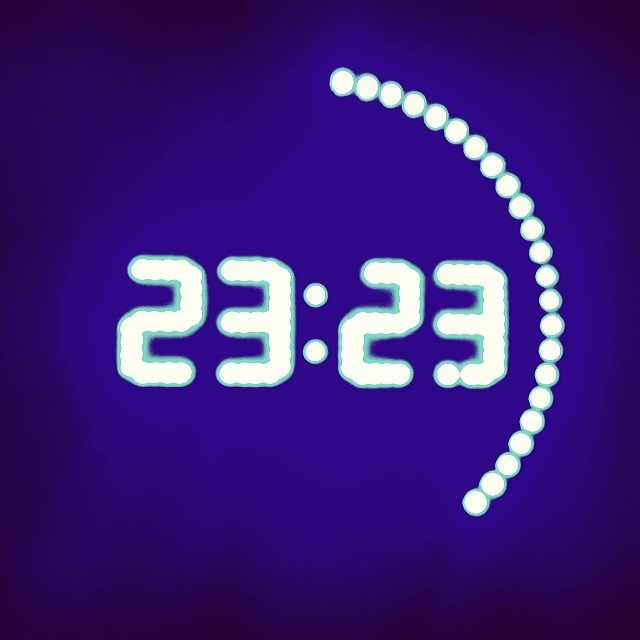This photograph showcases a vibrant blue digital clock displaying the time 23:23, which corresponds to 11:23 p.m. The time is presented in bright white illuminated digits that stand out against a dark royal blue background. Surrounding each minute of the hour, the clock features a series of bright white circles forming a circular shape on the right side. As the current time approaches 11:30, these luminous circles nearly complete a semicircle around the clock face, indicating the minutes elapsed in the hour. The scene is further enhanced by a gradient effect, with the blue hue transitioning from a lighter shade in the center to a dark navy blue around the photograph's edges, creating a visually appealing depth.